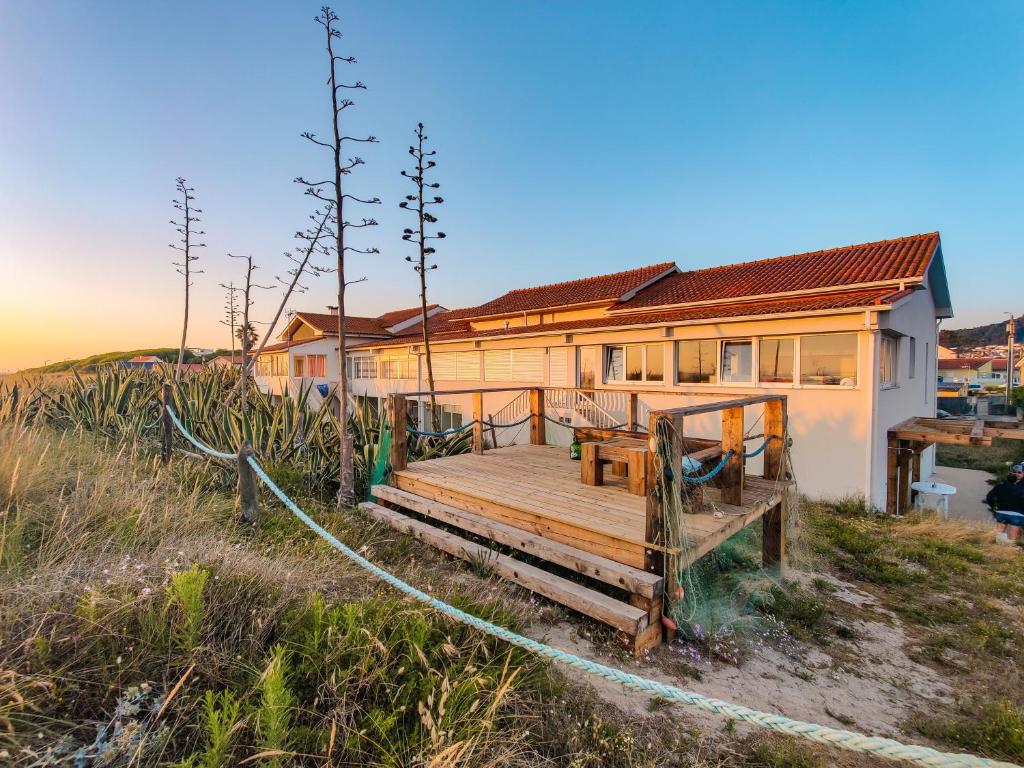This detailed image depicts a single-level, sand-colored house, possibly located in a desert or arid area, characterized by its reddish-brown or burnt orange roof, made from either clay or metal tiles. The house is adorned with numerous small windows across the front and features a small deck with two steps leading up to it. Surrounding the house is an array of plant life, including green and aloe plants, alongside sparse trees that appear to have buds but no leaves, hinting at a seasonal transition. In the background, another structure, resembling a barn with a rusted metal roof, can be faintly seen. There's also a rope fence adding a rustic charm to the scene. The sky above is clear with a rich blue hue and the lighting suggests it might be close to sunset, with brighter light focused on the left side. The overall scene is serene with no human or animal presence and no visible text, set against a backdrop of distant houses, hills, and possibly a mountain.